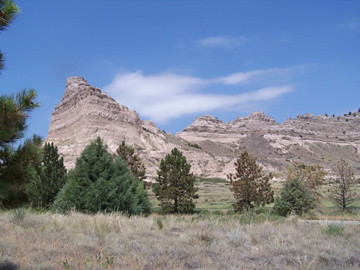This is a detailed photograph showcasing a serene and rugged natural landscape, likely taken in a mountainous region such as Colorado or Montana. The foreground features a mixture of dried and green-beige grass, punctuated by various trees that are predominantly evergreen. Among them, some trees exhibit signs of seasonal change with leaves browning, and there are even a few trees without leaves at all. The mid-ground displays an array of spaced-out pine trees, reminiscent of wild Christmas trees. Stretching across the background, there are imposing light gray and tan cliffs, their sheer and weathered surfaces starkly devoid of vegetation. Notably, some green bushes can be spotted on the right side of these cliffs. The top third of the image is dominated by a clear, bright blue sky, accented by a single, elongated white cloud that stretches horizontally across the scene, adding a dynamic yet tranquil touch to the composition. The absence of human elements accentuates the raw and untouched beauty of this picturesque outdoor setting.